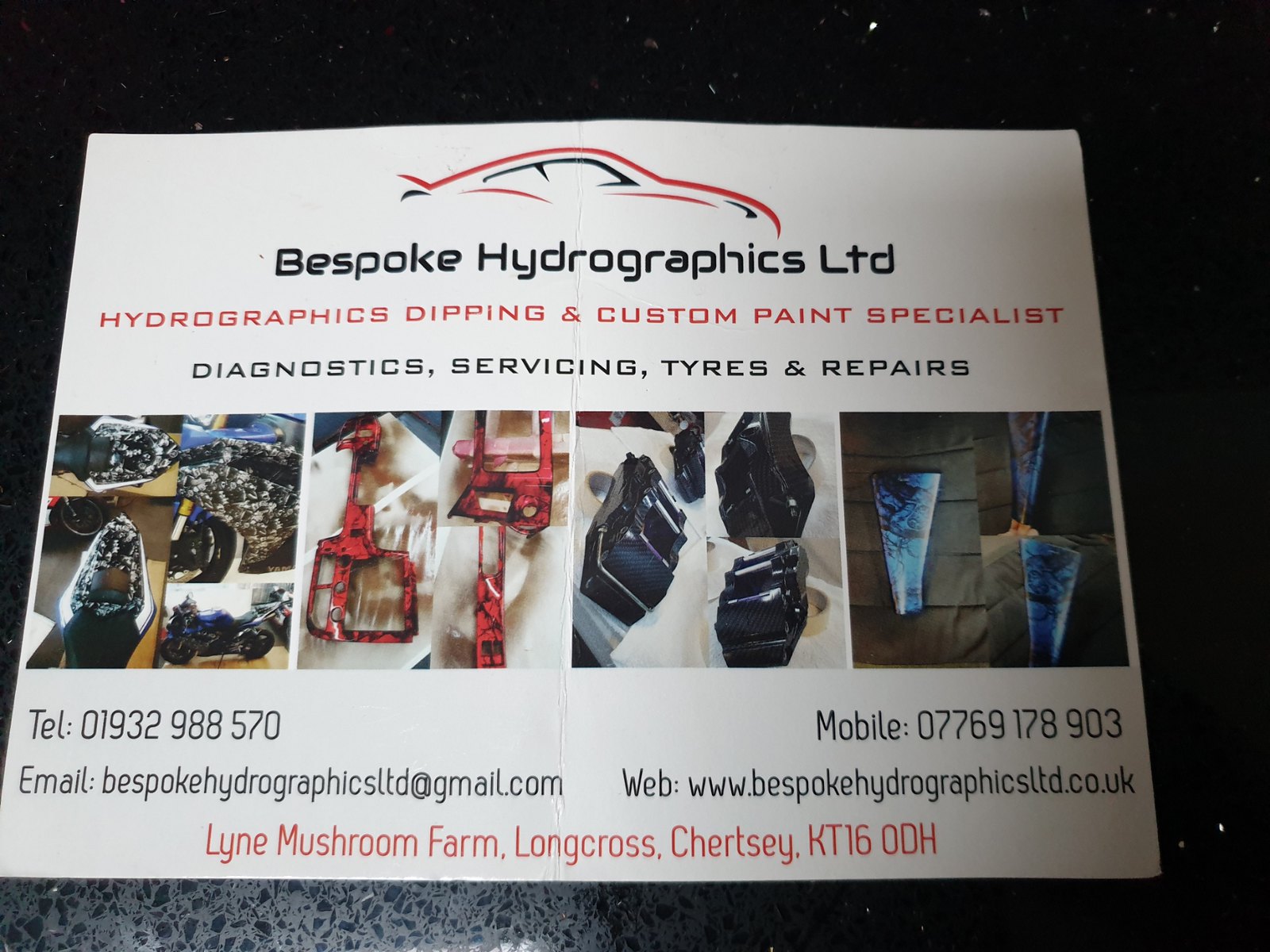The image features a large square with a solid black background, speckled sparsely with white and dark gray especially towards the bottom. Centrally positioned on this surface is a large, rectangular white poster board. At the top of the poster is a minimalistic illustration of a car, followed by the text "Bespoke Hydrographics Limited" in black. Just below this, in red text, it reads "Hydrographics Dipping and Custom Paint Specialists." Continuing in black text, there is information about "Diagnostics Servicing, Tires, TYRES and Repairs." Beneath these headers, there are four square sections, each containing images showcasing various hydro dipped products: a motorcycle tank, pedals, machinery, and another motorcycle part. At the bottom left, the contact details include a telephone number 01-932-988-570, and an email address bespokehydrographicsltd@gmail.com. To the right, there's an additional mobile phone number 07769 178903 and a website URL www.bespokehydrographicsltd.co.uk. Centered at the very bottom in red text, it states: "Line LYNE Mushroom Farm, Long Cross, Chertsey, KT160DH."